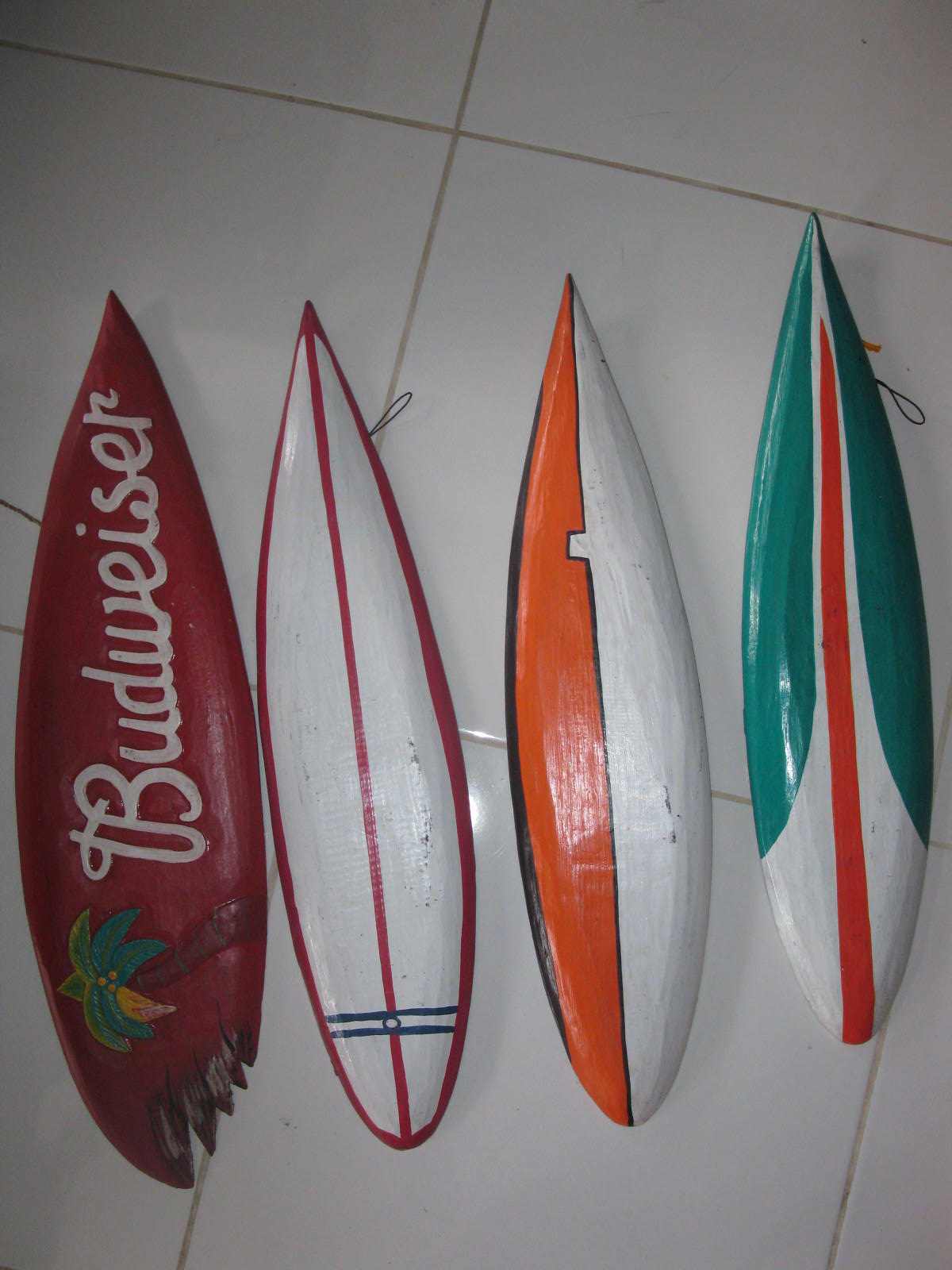The image captures a bird's-eye view of a white tiled floor, potentially marble, featuring four miniature surfboards with unique designs laid side by side from left to right. The tiles are notably large, lending an expansive backdrop to the arrangement.

The surfboard on the far left is fully red with the word "Budweiser" written in white cursive accompanied by a palm tree graphic. It also appears to have "teeth marks" or a jagged edge, suggesting a design element meant to mimic shark bites. Next to it, the second surfboard is primarily white, edged with a thin red border. It features a horizontal blue stripe near the base and a blue circle at its center. The third surfboard is divided into an orange and white half, complemented by a black outline. The final surfboard on the far right is predominantly white, adorned with a vertical orange-red stripe and flanked by dark teal sections.

These surfboards are notably small, hinting at their decorative purpose, possibly for use in an establishment or shop rather than functional surfing equipment.